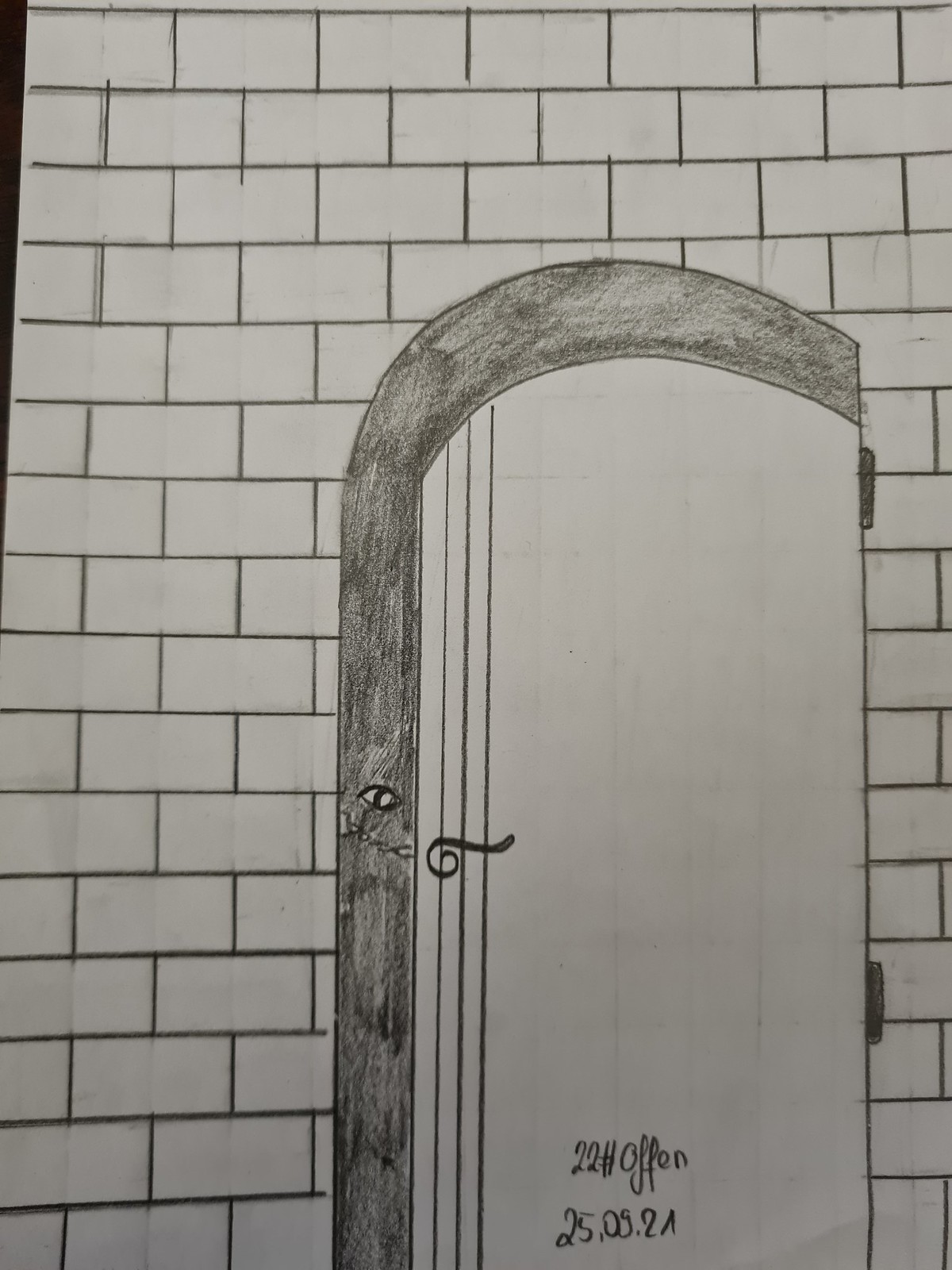This monochromatic pencil drawing, meticulously rendered on stark white paper, captures a detailed scene of a brick wall composed of horizontal, evenly laid bricks. The composition stretches almost across the entire frame of the photograph, with a narrow black border peeking through at the upper left corner. Dominating the right and lower half of the drawing is a prominently featured arched door. This wooden door, affixed with two visible hinges on its right, is slightly ajar, revealing a narrow, darkened crack along its top and left edges. A chain door lock restricts the door’s further opening, adding to the scene's subtle tension. Peeping through the darkness just above the chain lock is a small, eerie eye with a slit pupil. Adjacent to the chain lock on the door's right side is a spiral lever-shaped door handle, completing the intricate details of this thought-provoking and slightly unsettling piece.